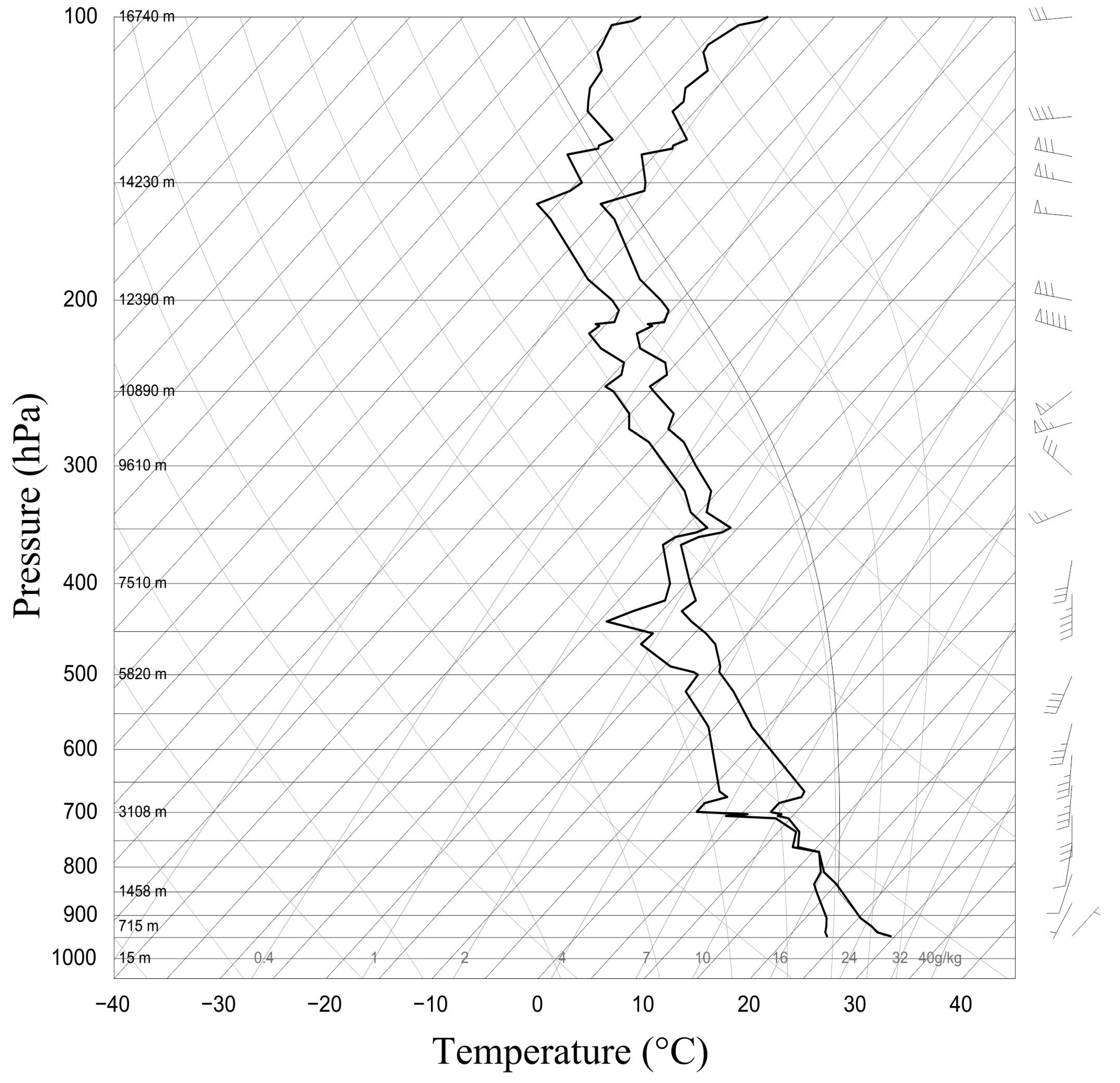This detailed graph measures pressure (in hPa) against temperature (in degrees Celsius). The y-axis on the left ranges from 1,000 hPa at the bottom to 100 hPa at the top, with more dense increments at higher pressures and broader increments at lower pressures. Additionally, the y-axis includes a secondary measurement on the right side, ranging from 15M to 16,740M in irregular intervals. The x-axis at the bottom displays temperature, ranging from -40°C to 40°C in 10-degree increments. 

A distinctive feature of the graph is two jagged black lines traversing from just above the center at the top towards the bottom right corner, indicating the relationship between pressure and temperature. The graph also contains a loose grid-like pattern comprised of diagonal and some curved gray lines. On the far right, numerous symbols resembling line segments with shorter lines attached at various angles add more detail.

The graph predominantly uses black lines over a white background with light gray grid lines, making it a likely candidate for a scientific textbook illustration. Its meticulous layout and comprehensive representation of data make it helpful for understanding the interplay between temperature and pressure.